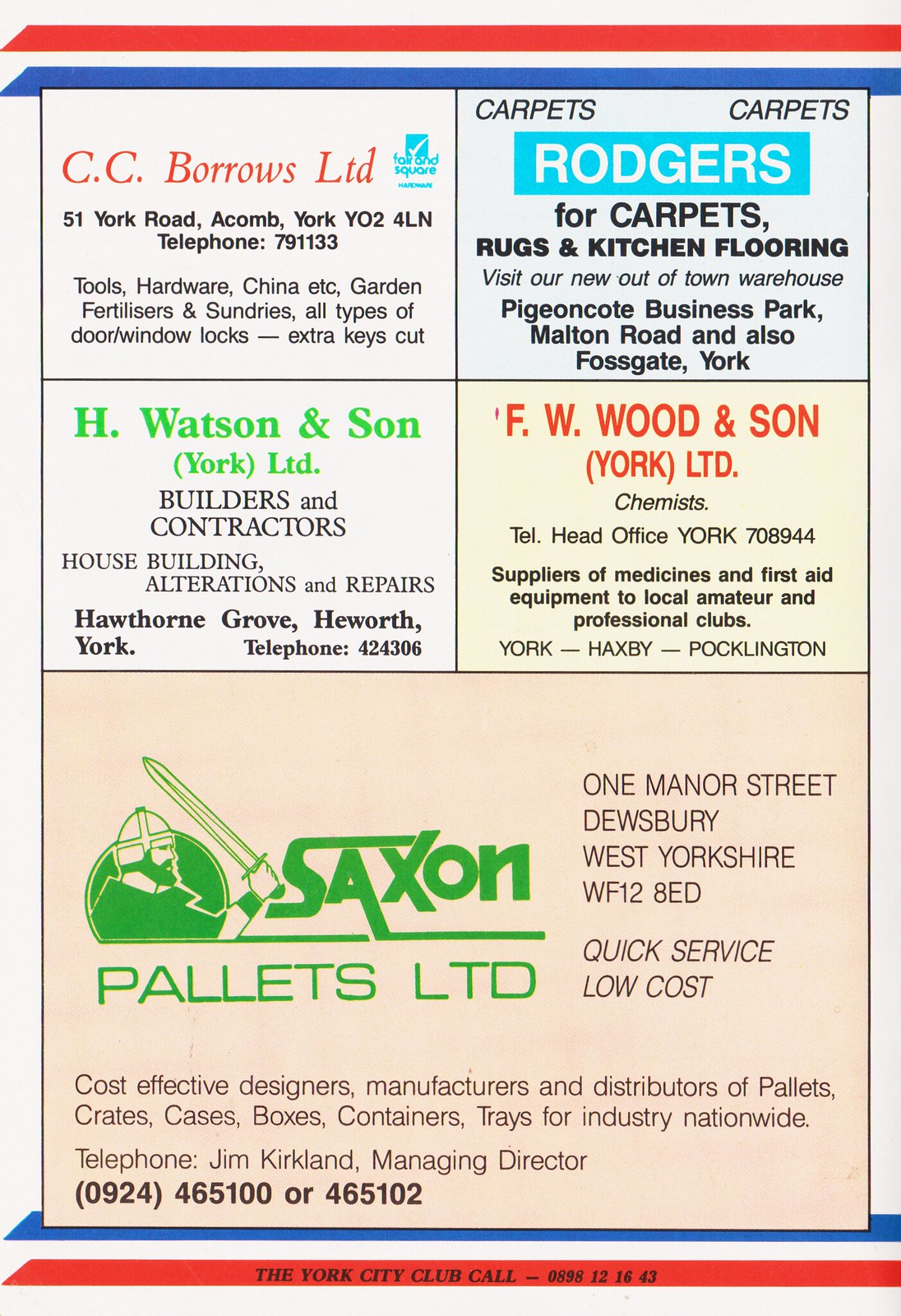The image depicts a scan of a magazine page or pamphlet on an off-white background with a border of red and blue stripes. The page is segmented into five advertisements: the upper half contains four equally-sized advertisements, while the bottom half features one large advertisement. The sections are divided by horizontal lines and share a light blue background.

**Top Left Advertisement:** 
- **Business:** CC Burroughs, LTD
- **Details:** 51 York Road, Acom, York Y024LN, Telephone: 791133
- **Products/Services:** Tools, Hardware, China, Garden Fertilizers and Sundries, Door and Window Locks, Extra Keys

**Top Right Advertisement:** 
- **Headline:** "Rogers for Carpets, Rugs and Kitchen Flooring" 
- **Details:** Visit our new out-of-town warehouse at Pigeon Cot Business Park, Malton Road and also Fossgate, York

**Bottom Right Advertisement in Top Section:** 
- **Business:** H. Watson and Son, York LTD
- **Details:** Builders and Contractors, House Builders, Alterations and Repairs, Hawthorne Grove, Heworth, York, Telephone: 424306

**Bottom Left Advertisement in Top Section:**
- **Business:** F.W. Wood and Sons, York LTD
- **Details:** Chemists, Telephone Head Office, York: 708944
- **Specialization:** Suppliers of Medicine and First Aid Equipment to Local Amateur and Professional Clubs in York, Haxby, and Pocklington

**Large Bottom Advertisement:**
- **Business:** Saxon Pallets LTD
- **Logo:** Green logo featuring a man in a medieval helmet with a sword
- **Details:** One Manor Street, Dewsbury, West Yorkshire, WF128ED
- **Services:** Quick Service, Low Cost, Cost-Effective Design, Manufacture, and Distribution of Pallets, Crates, Cases, Boxes, Containers, and Trays for Industry Nationwide
- **Contact:** Jim Kirkland, Managing Director, Telephone: 0924-465100 or 465102

At the very bottom of the page, in black text on the red line, there's an advertisement for York City Club, Call 0898-121643.